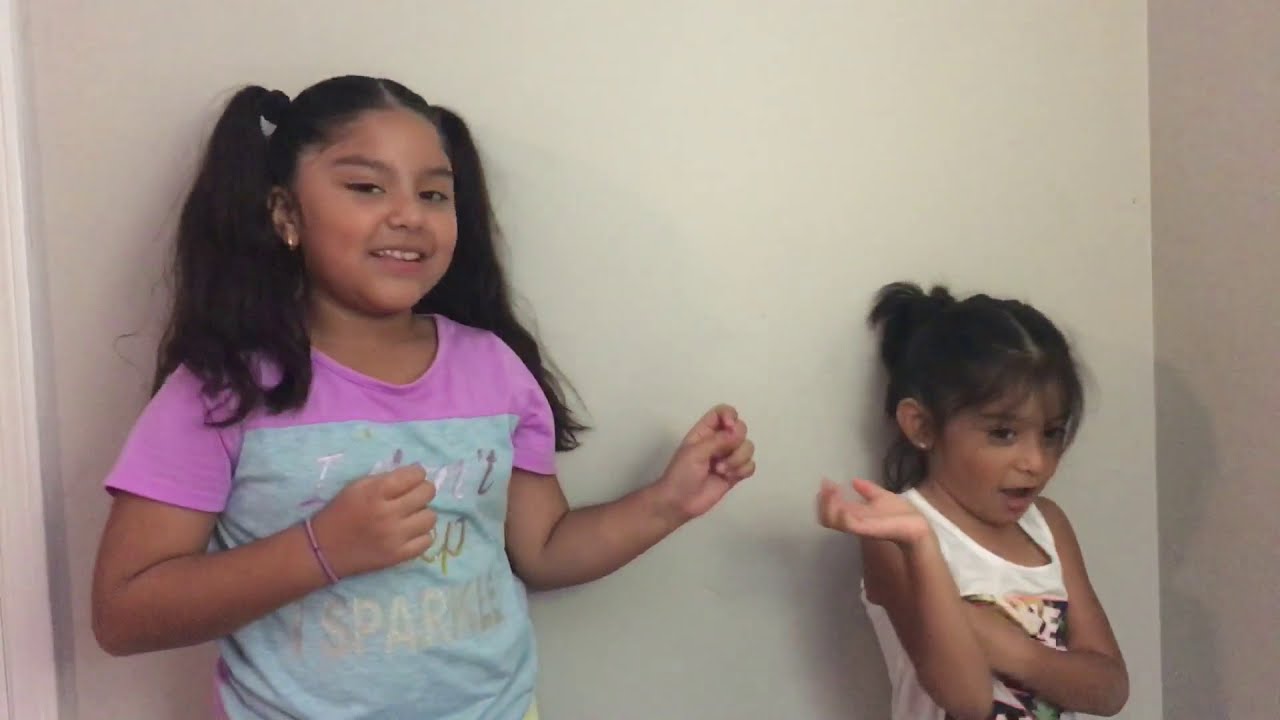The image portrays two Hispanic girls standing against a white wall. The picture is a horizontal rectangle and shows the girls from the waist up. The backdrop features an intersecting white wall with a darker brown shade on one side. Both girls have a slightly tan complexion and are adorned with small earrings. 

The girl on the left is the taller of the two, with long black hair styled into pigtails, each tied up and falling to her collar. She is dressed in a vibrant pink and blue t-shirt with the word "Sparkle" printed across it. Her arms are bent at the elbows, with her hands fisted and angled to the sides of her body, and she is smiling confidently at the camera. She also sports a small purple bracelet on one wrist.

The shorter girl on the right has her hair pulled back into a ponytail, with bangs framing her forehead to her eyebrows. She is wearing a white sleeveless tank top with a graphic, possibly characters, on it. Her left arm is crossed over her chest, and her right arm is bent at the elbow with her hand palm-up, as if in mid-gesture. Her mouth is open, giving the impression she might be speaking or expressing surprise.

The setting and the girls' animated poses suggest they could be performing, perhaps for a video or podcast, indicating an element of playfulness and engagement between them. Their similar appearances hint they might be sisters.